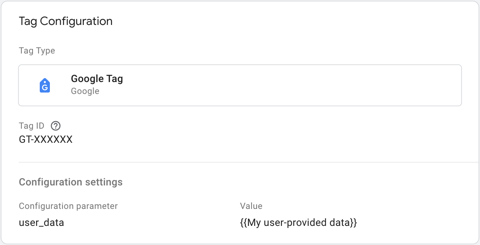The image showcases the detailed layout of a tag configuration interface. In the top left corner, there's the section labeled "Tag Configuration." On the left side, there's a dropdown or menu indicating different "Tag Types." Adjacent to this, there's a square box labeled "Blue Tag." Below this, there's another box titled "Google Tag," with the word "Google" clearly visible above it. Following this, the "Tag ID" is displayed, showing a code in the format "GT-XXXXX."

Next to the "Tag ID," there's an icon resembling a question mark, potentially for help or more information. Underneath this information, there's a line item for "Configuration Settings," detailing various parameters. One of these parameters is "user_data," next to which is a "Value" field. This field contains placeholder text in double brackets labeled "my user-provided data." The background of the entire interface is stark white, creating a clear and focused presentation.

Though the image appears slightly out of focus, we can still discern the structured arrangement of configuration settings and parameters, such as "user_data" and its corresponding value, indicating "my user-provided data." The edges of the image are clean and sharp, contributing to the overall neatness of the tag configuration layout.